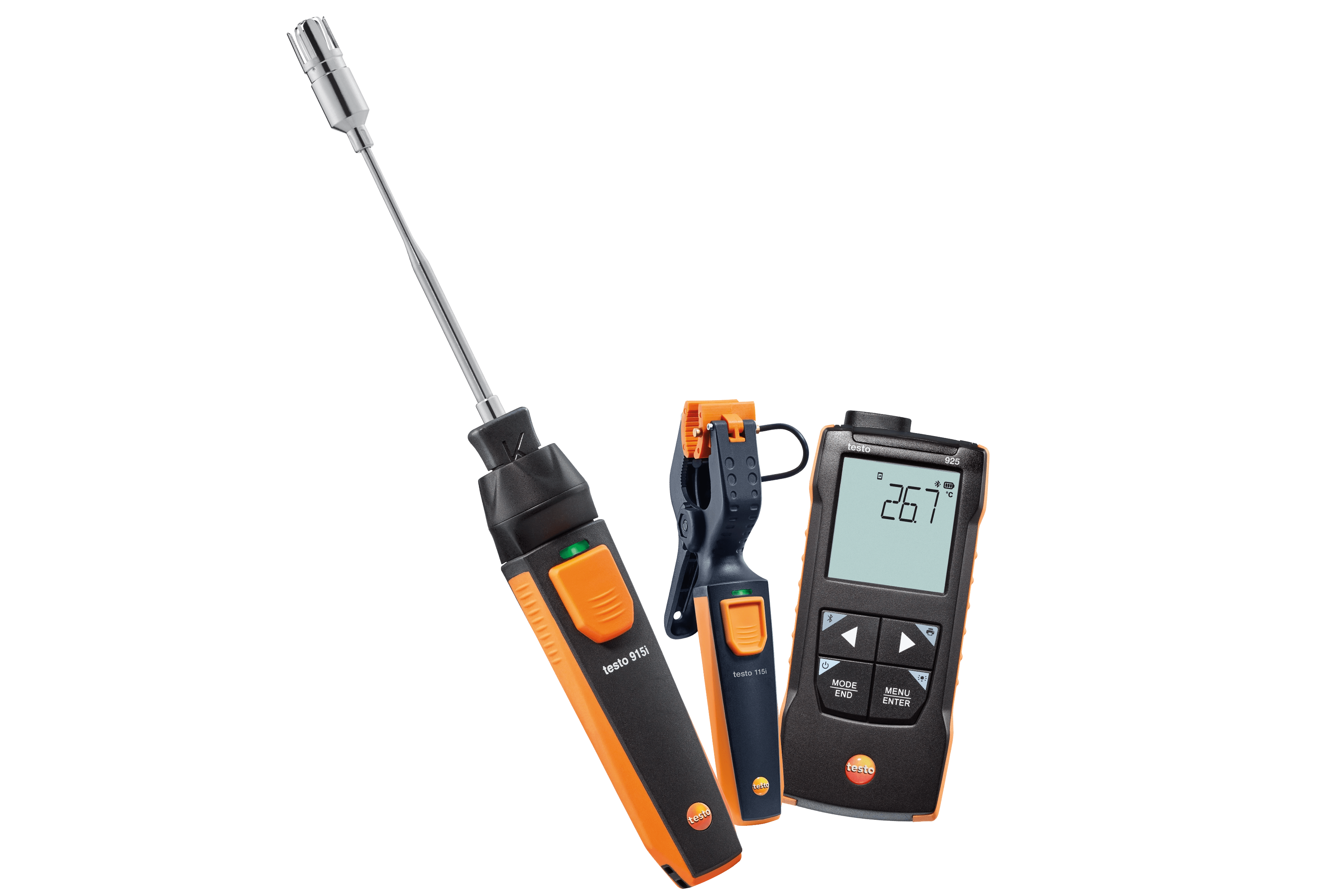The image showcases three distinct electronic tools against a white background. On the left, there is an electric screwdriver with an orange and black handle, featuring a large orange power button and a small green light above it. This tool connects to a silvery telescopic rod ending in a cylindrical knob. To the right, there is a pair of pliers with a matching orange and black handle, a serrated grip at the tips, and a small tube connecting the handles on the back. Further to the right, a handheld digital meter about the size of a cell phone is visible, sporting an LCD screen currently displaying "26.7" and four buttons arranged in a square pattern. Each of these tools shares a consistent design theme of black and orange, suggesting they are from the same manufacturer.